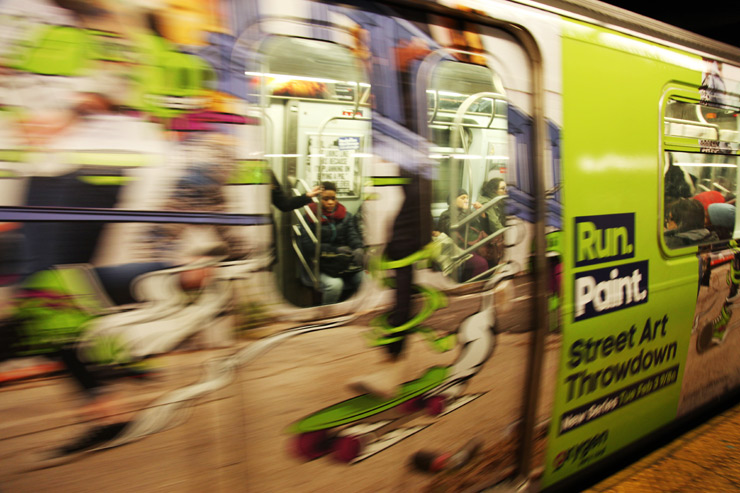A photograph captures a moving commuter train, wrapped in green artwork reminiscent of cartoonish figures, similar to a Ren and Stimpy aesthetic. The train's exterior features the text "Run, Paint, Street Art, Throwdown," suggesting a sponsored graffiti art project or a television series advertisement. The train's motion is evident from the blurred image, hinting at a fast shutter speed. Visible through the train windows are several passengers: an African-American woman sitting alone, another window shows a man and woman side by side, and the window closest to the viewer reveals the backs of several people, including a child in a blue beanie. All passengers appear dressed in warm clothing, suggesting it's fall or winter. The scene resembles an underground railway system, possibly the New York City subway, with dim interior lighting contrasted by the vibrant exterior.